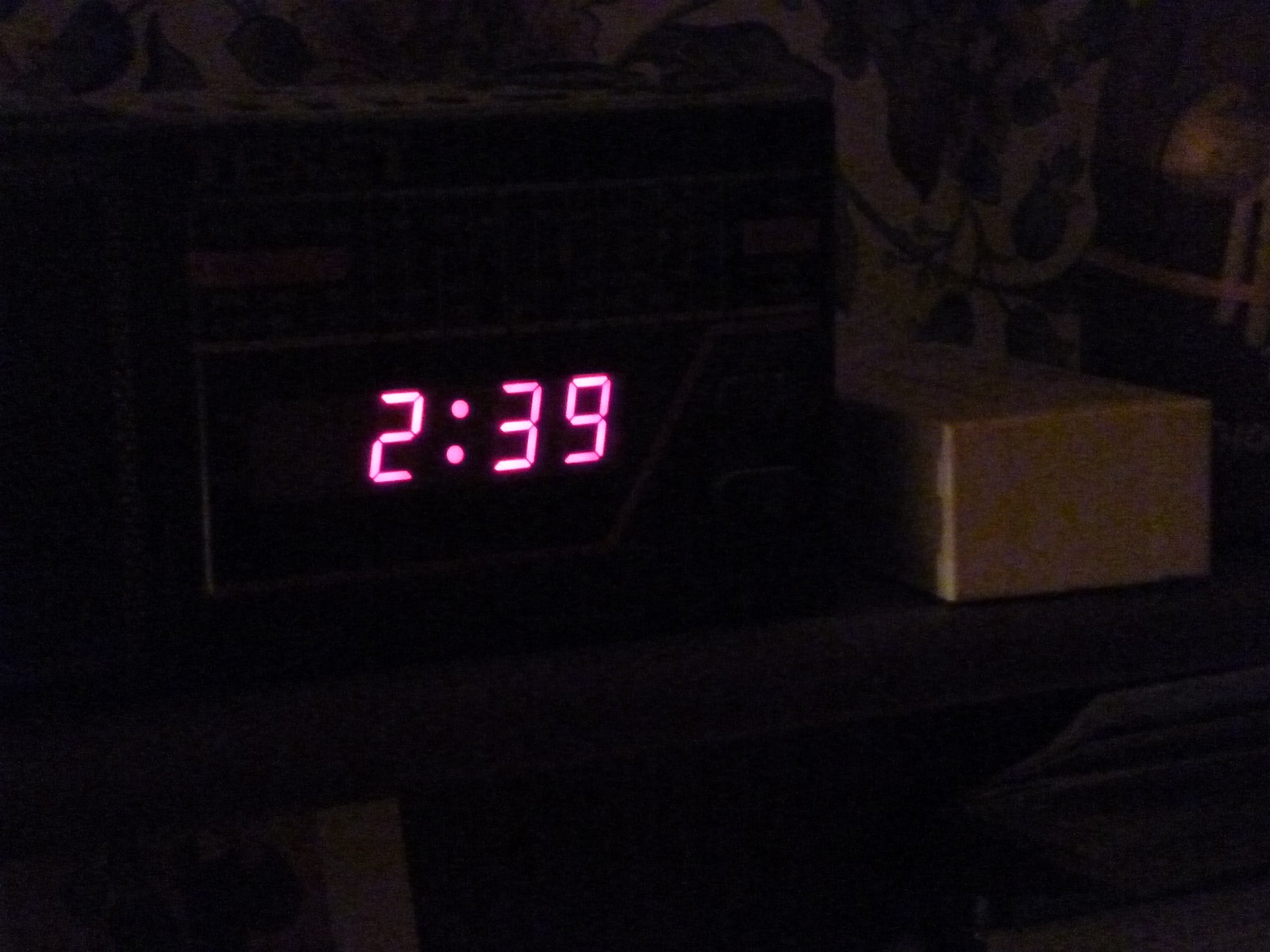The color photograph captures a very dark room, where the primary source of light emanates from a digital alarm clock displaying the time as 2:39 in hot pink digits. The clock, with its small buttons on top, rests on a shelf. To its right sits a small, unopened brown box. Behind the clock, the wall features a white background adorned with blue and yellow floral patterns. Below the shelf, the bottom of the image remains obscure, though the faint outlines suggest the presence of magazines or books stacked in the lower right corner, possibly resting on a very dark wooden table.